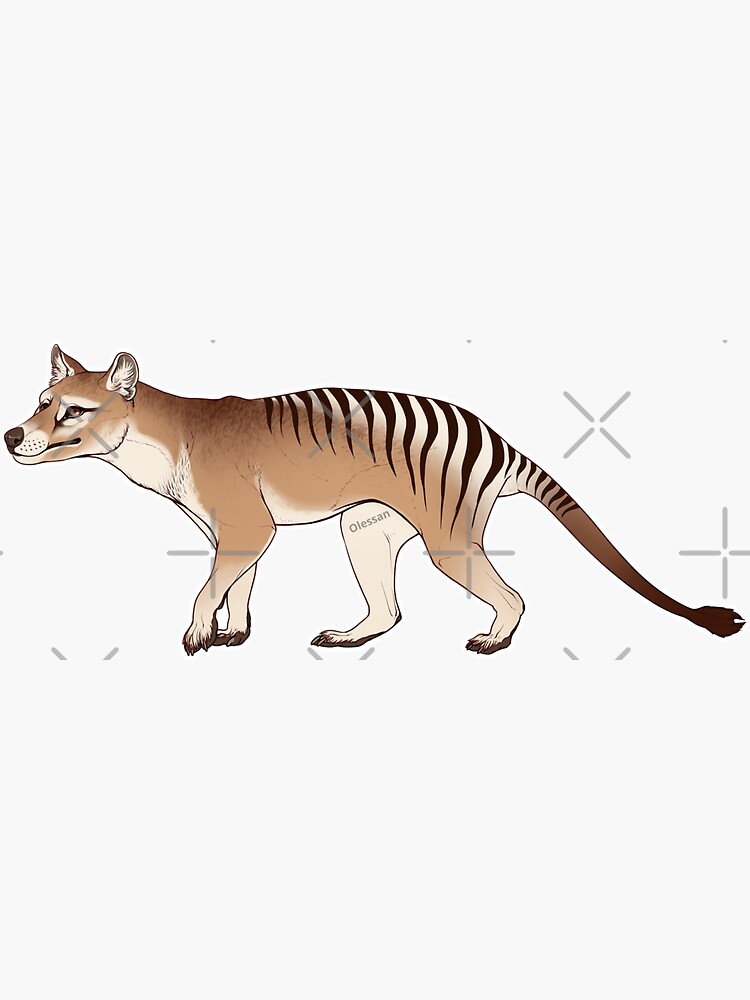This slightly vertical illustration depicts a Tasmanian tiger, drawn in profile and gazing towards the left. The animal, now extinct, is depicted with a dog-like head and ears, as well as similarly shaped limbs. Its back displays distinct stripes, while its tail is characterized by a long, sleek form ending in a tuft. The color palette includes a medium brown-tan for its upper body, transitioning to a lighter tan on the underbelly. The image is marked with watermarks that state "oh the sun," and interspersed with X's and plus marks.